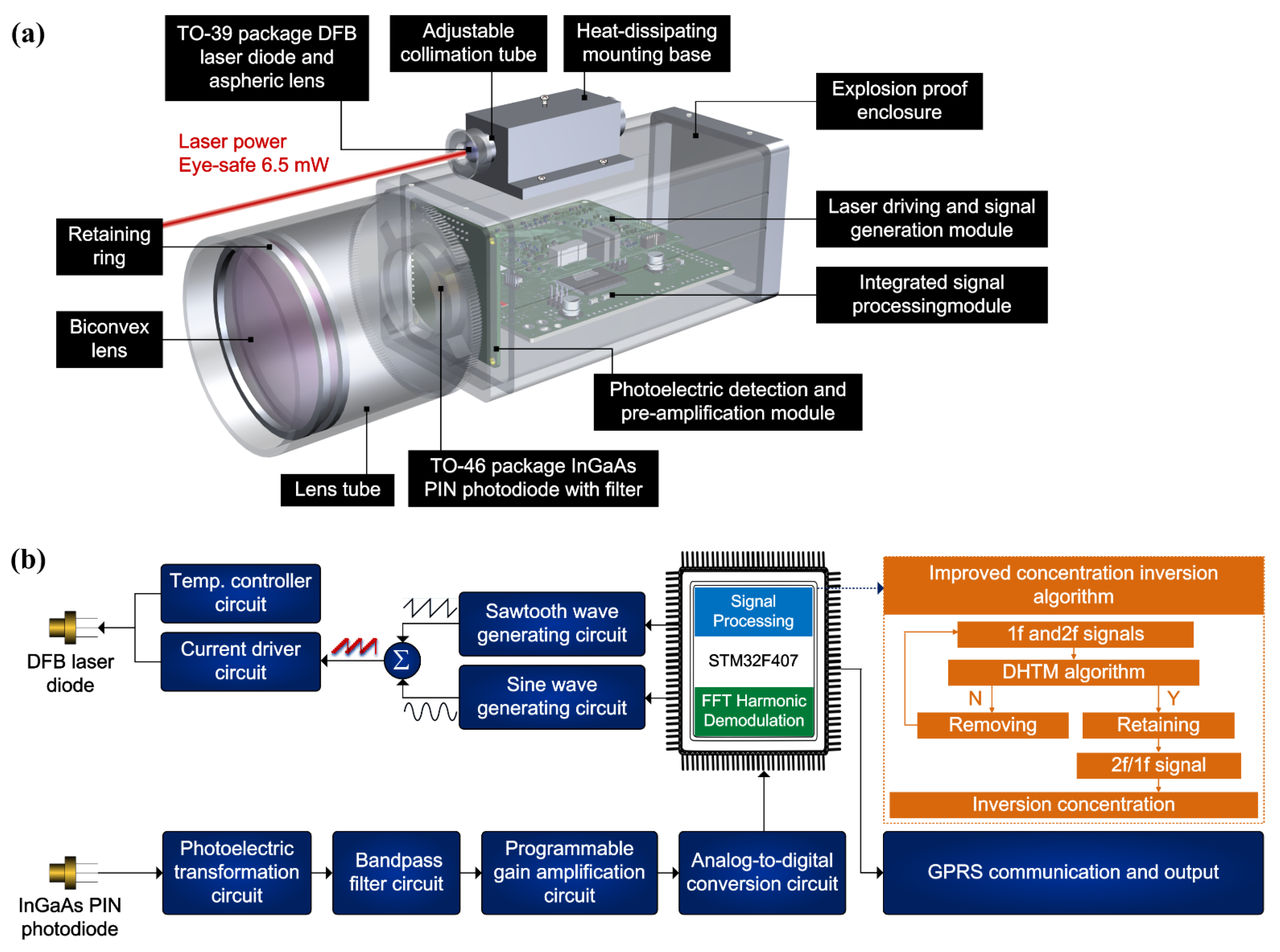The image portrays a detailed diagram explaining the workings of a laser-based device, likely a measurement or scanning tool. At the top, labeled "A," is an intricate terrarium-like tank featuring a camera, a cylinder, and a series of black rectangles with white text pointing to various components. These labels include "bi-convex lens," "retaining ring," "laser power: eye safe, 6.5 nw," "239 package DFB laser," "adjustable lens tube," and "heat dissipating mounting base," among others.

Below, labeled "B," is a secondary diagram showcasing additional parts. This section highlights a gold cylinder atop a wider circle, flanked by blue rectangles with white, curved-edge text. Black rectangles with internal white sections detail further internal components, with sections colored blue, white, and green. Additional blue rectangles with white text describe more specifics.

In the bottom right, orange-outlined rectangles with white text offer further descriptions, accompanied by yet another blue rectangle with curved edges and white writing. Collectively, the diagram provides a comprehensive breakdown of the device's components and their functions, including "laser diode," "aspheric lens," "retaining ring," "biometric lens," and "lens tube," and details various processes like "NGAAS pin photodiode," "photoelectric transformation circuit," "bandpass filter circuit," "programmable gain amplification circuit," and "analog to digital conversion circuit."